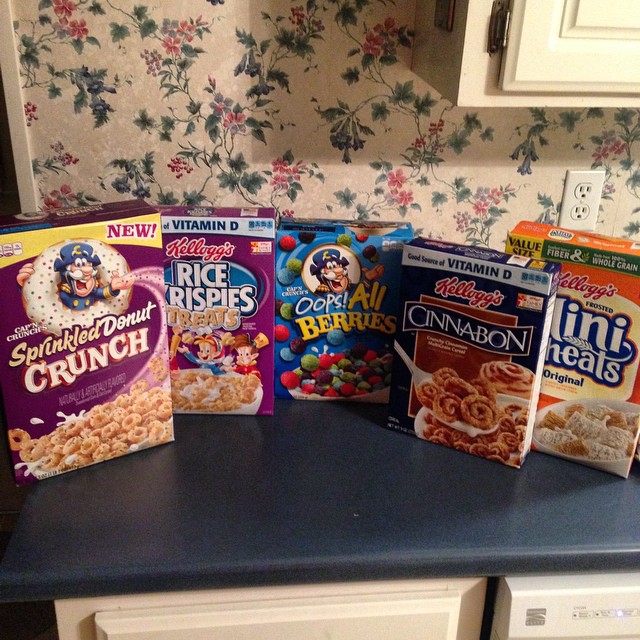This photograph, taken in a kitchen, features five vibrant cereal boxes neatly lined up from left to right on a dark blue countertop. The countertop is part of a kitchen setup with white wooden drawers below and a white cabinet visible in the top left corner. The backsplash is adorned with vintage-style wallpaper featuring red flowers with green stems and leaves, and a white outlet is noticeable on the right side. 

The cereal boxes are:

1. Cap'n Crunch's Sprinkle Donut Crunch in a purple box, showcasing the Cap'n popping through a doughnut with pink swirls and a bowl of the cereal below.
2. Kellogg's Rice Krispie Treats in a similarly purple box, featuring Snap, Crackle, and Pop inspecting a bowl of their cereal.
3. Cap'n Crunch's Oops! All Berries in a blue box, depicting a cascade of colorful berries into a bowl of milk.
4. Kellogg's Cinnabon in a dark blue box, showing miniature cinnamon rolls in a bowl, some lifted by a spoon.
5. Kellogg's Frosted Mini-Wheats Original in a bright orange box, displaying mini-wheats with frosted tops in a bowl of milk.

The scene captures the rich colors and detailed graphics of these brightly packaged, sugary cereals against the backdrop of a well-used, charmingly patterned kitchen.